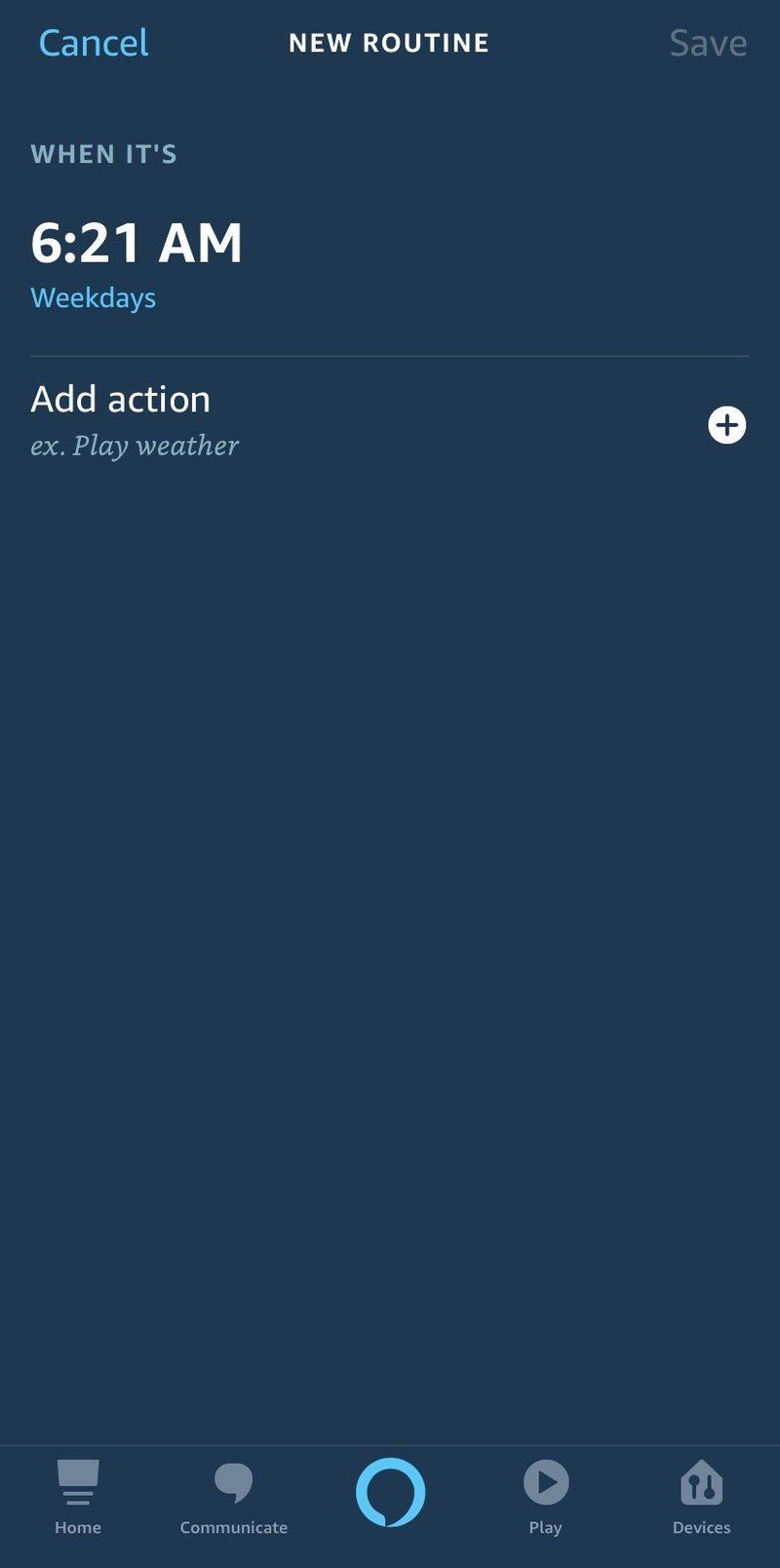A screen displays a black interface, likely a note-taking or task management device. At the top, a blue "Cancel" button is situated on the left, with the title "New Routine" centered in white. To the right, a "Save" button is visible but grayed out. Below this header, the screen features sections with black backgrounds and text in varying colors. The first section reads "When it's 6:21 a.m." in white, followed by "weekdays" in gray.

A subtle blue line divides the screen from the next section which prompts the user to "Add Action." An example action, "ex. play weather," is given in gray text, alongside a button for adding more actions. The rest of the screen remains blank with a solid black background.

At the bottom of the screen, there are five icons: a mute symbol, a thought bubble labeled "Communicate," a blue circle that is almost complete (likely indicating activation), a play symbol, and an icon for "Devices." The blue circle stands out as it suggests an active state, contrasting with the other, likely inactive, icons.